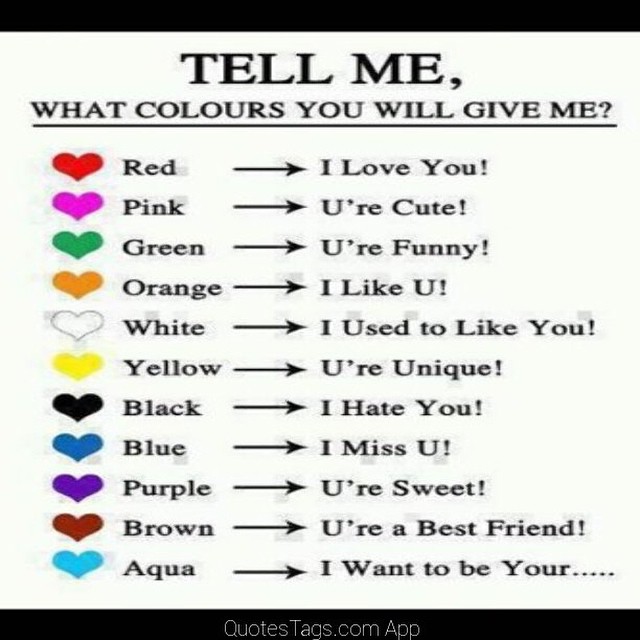This image, seemingly sourced from a website or the internet, showcases a chart with a black bar at the top and another black bar at the bottom labeled "QuotesTags.com App." The focal point of the image is a list of questions and corresponding answers indicated by differently colored hearts arrayed vertically on the left side. The black text at the top of the image reads, "Tell me, what colors will you give me?" 

Each heart color is associated with a specific sentiment:
- Red heart with an arrow pointing to "I love you."
- Pink heart with an arrow pointing to "You're cute."
- Green heart with an arrow pointing to "You're funny."
- Orange heart with an arrow pointing to "I like you."
- White heart with an arrow pointing to "I used to like you."
- Yellow heart with an arrow pointing to "You're unique."
- Black heart with an arrow pointing to "I hate you."
- Blue heart with an arrow pointing to "I miss you."
- Purple heart with an arrow pointing to "You're sweet."
- Brown heart with an arrow pointing to "You're a best friend."
- Aqua heart with an arrow pointing to "I want to be your... (ellipsis)"

The chart conveys a range of feelings, typically used in a playful, social media context to prompt responses about which colored hearts would be given to someone based on their relationships or feelings towards that person.